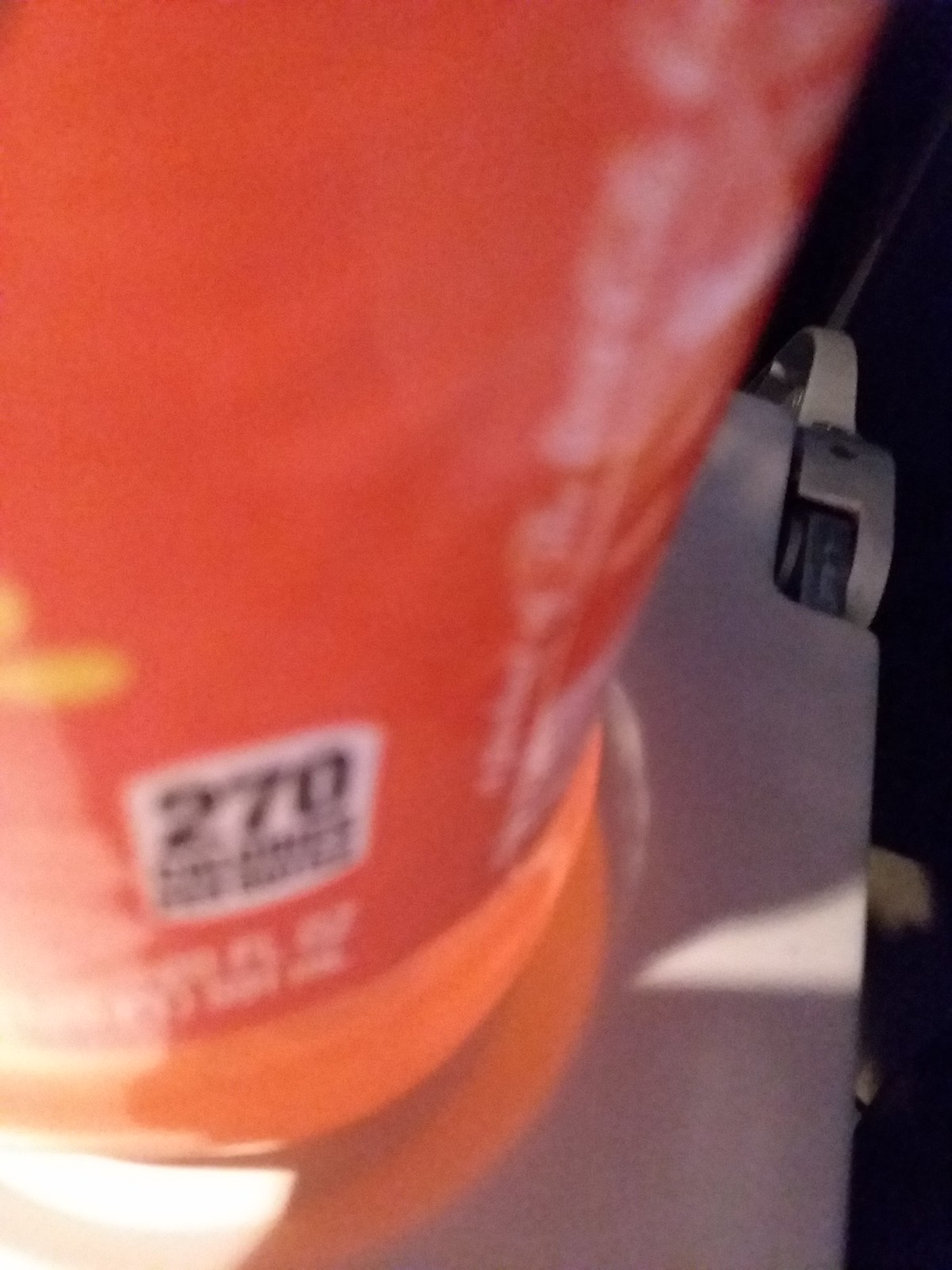This close-up photograph features a blurry image of a bottle, predominantly red in color with an orange bottom. A white rectangular label with black text reading "270" is visible near the bottom of the bottle, although additional text surrounding it is indistinct due to the blurriness. The red bottle appears to be placed on a grayish, machinery-like surface, possibly due to the presence of elements resembling a wheel track or a lamp in the background. On the right side of the bottle, there is vertical white text, likely a reflection, contrasting the otherwise vivid red and orange hues. The orange section suggests it might contain an orange liquid, possibly hinting at the bottle being a drink, likely an energy beverage like Gatorade. The combination of reflections and the photographic blur enhances the complexity of the image.